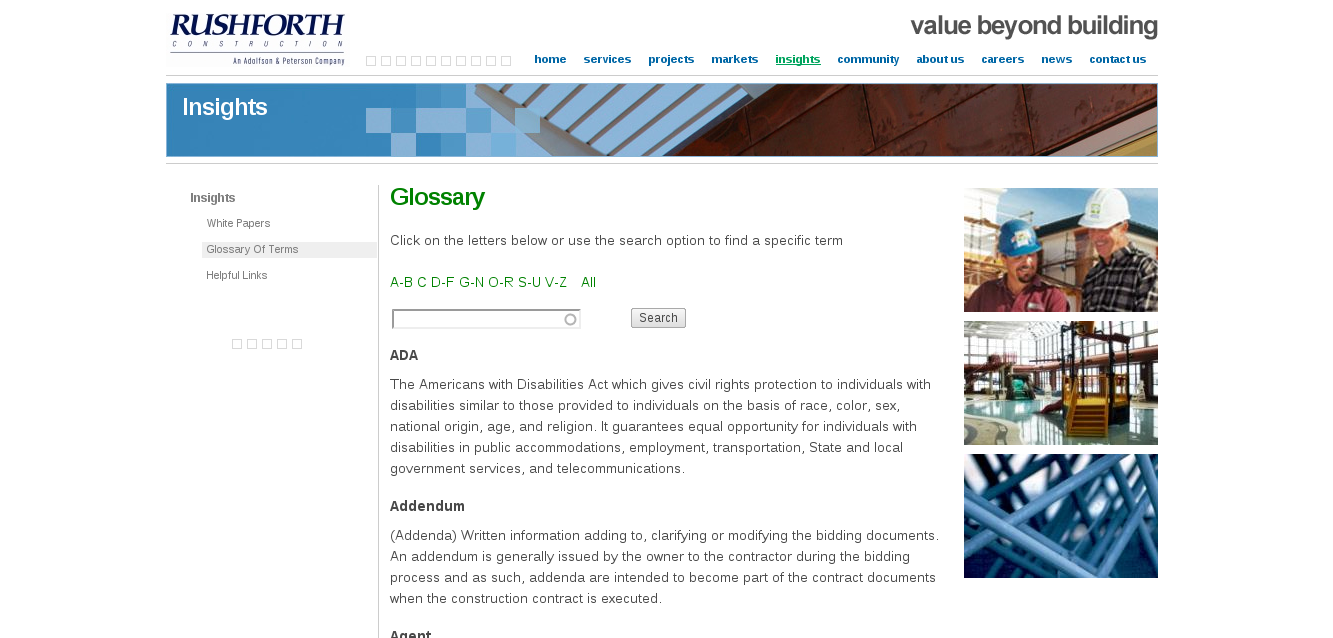This screenshot captures the glossary page of a website associated with Rushforth Construction. In the top left corner, the branded title "Rushforth" is prominently displayed, with "Construction" written in smaller text directly below it. A thin horizontal line underscores these elements, emphasizing the branding.

To the right, a top navigation bar offers various menu options: Home, Services, Projects, Markets, Insights, Community, About Us, Careers, News, and Contact Us. All buttons are highlighted in blue, except for "Insights," which stands out in green and features a matching underline, indicating the current page.

Adjacent to the navigation bar, the motto "Value Beyond Building" is subtly placed. Below this slogan, a header image labeled "Insights" appears, displaying the intricate details of a ceiling, which adds a visual element that complements the content focus.

Further down the page, a sidebar titled "Insights" is visible. Underneath this section header, links to subsections, such as Woodpapers, Glossary, Terms, and potentially other useful links, are listed, allowing for easy navigation within the Insights section.